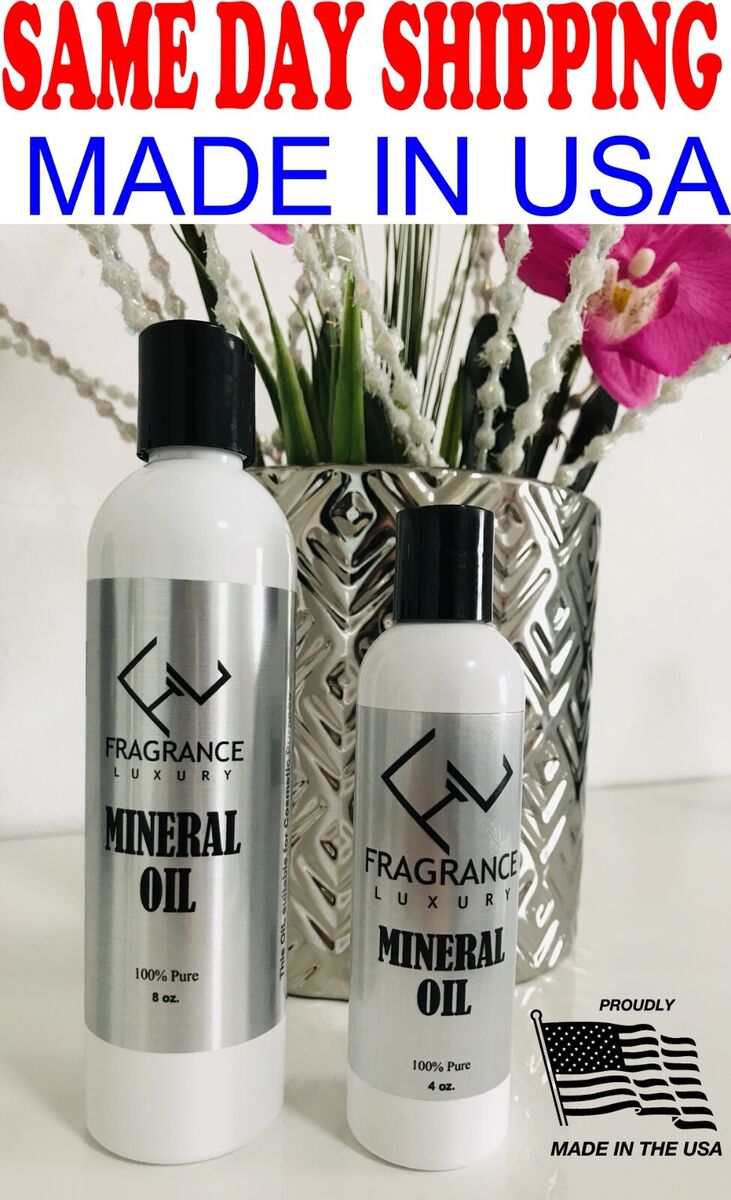This detailed advertisement photograph showcases two elegant, cylindrical plastic bottles of fragrance luxury mineral oil, 100% pure, positioned side by side on a pristine white countertop. The smaller bottle holds 4 ounces, while the larger contains 8 ounces, sporting sleek black caps and silver foil labels. Prominently featured on the top of the image in bold red and blue text are the phrases, "Same Day Shipping" and "Made in USA", emphasizing convenience and national pride. Complementing the minimalist design of the bottles is a sophisticated silver vase with a geometric impressed design, enhancing the luxury theme. The vase contains green faux leaves, white fillers, and a striking large pink faux hibiscus, adding an element of elegance and vibrancy to the scene. On the lower right hand corner, a logo proudly proclaims the product's American origin with an American flag icon and the statement, "Proudly Made in the USA". The advertisement balances aesthetic appeal and informative details, promoting the mineral oil as a premium, domestically made product.